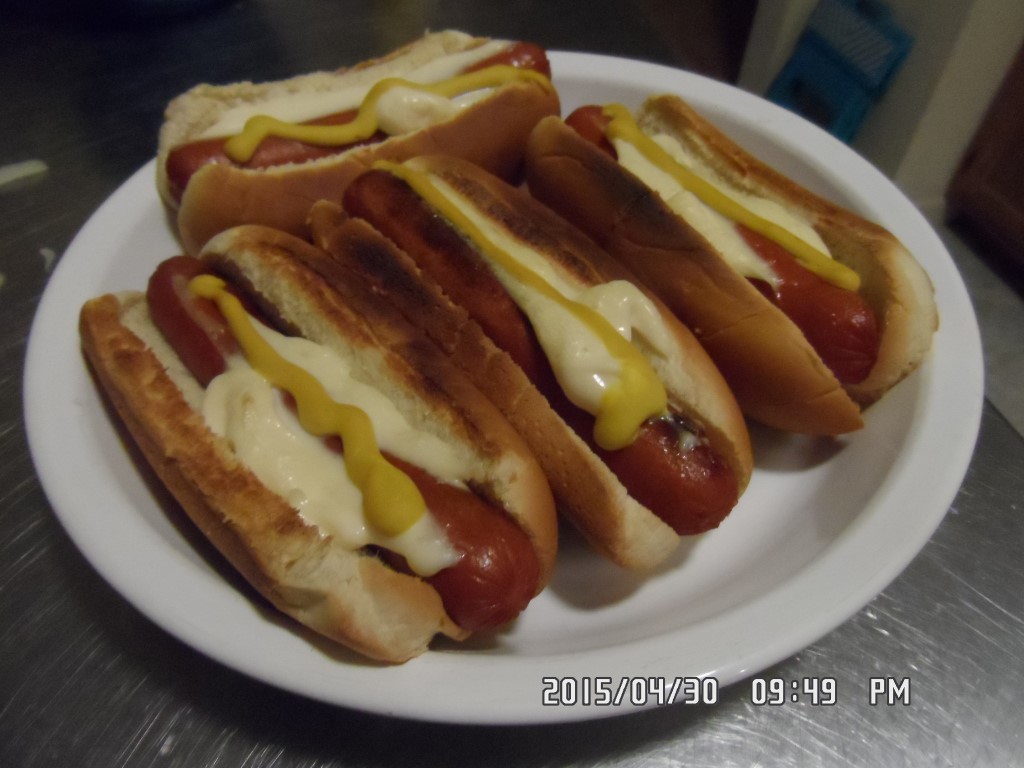In this image taken on April 30th, 2015, at 9:49 PM, we see four hot dogs meticulously arranged on a white ceramic plate, placed atop a grayish, stainless steel table. The picture is somewhat zoomed in, focusing mainly on the hot dogs, which are encased in browned and toasted buns that exhibit hints of almost burnt spots. Each hot dog is garnished with a stripe of mustard running lengthwise and mayonnaise applied along the sides. Some descriptions suggest the possible presence of melted cheese. The hot dogs and buns appear freshly cooked, showing a char that adds to their allure. Three hot dogs are aligned parallel to each other, while the fourth is oriented perpendicularly at the end of the plate, likely due to space constraints. The background features faint, blurred elements of what seems like furniture, adding a homely touch to the setting.